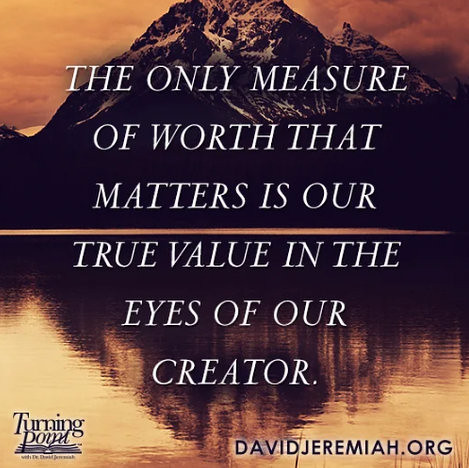This square image, reminiscent of a motivational or social media post, serves as an advertisement for a religious service. The backdrop showcases a stunning mountain peak with hints of snow, set against a cloudy sky tinged with an orangish-gold hue, suggesting a serene sunset. Below the mountain, a tranquil lake mirrors the peak and sky, creating a blurry but captivating reflection. The text, written in white and spread across the mountain and lake, reads: "The only measure of worth that matters is our true value in the eyes of our creator." In the lower-left corner, there's a logo of an open book accompanied by the words "Turning Point," and in the lower-right corner, the website "DavidJeremiah.org" is displayed.